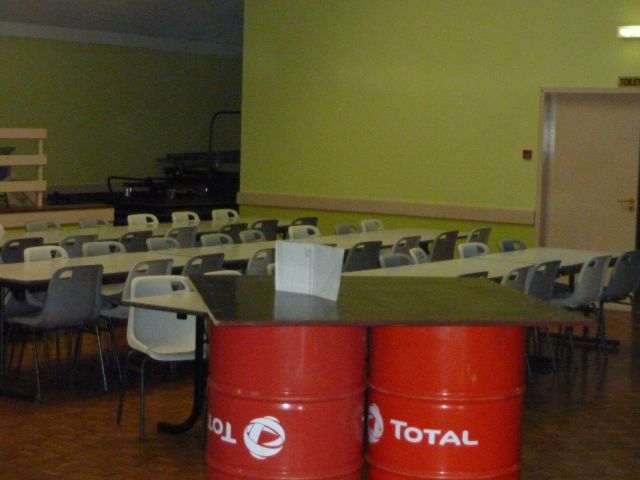The image is a color photograph taken inside a school cafeteria characterized by large, yellow walls—light yellow at the top, transitioning to a slightly darker yellow below the chair rail. The room is illuminated by fluorescent lighting visible in the upper right corner, and an exit sign is mounted above a door on the right side. The cafeteria is furnished with three rows of long white tables, each flanked by approximately eight molded plastic chairs commonly found in elementary schools. All the chairs are identical, cheap-looking, and slightly hard. In the foreground, two red 55-gallon drums, both labeled with the word "TOTAL" in white lettering along with a globe-like ribbon logo, serve as makeshift supports for a large, dark-colored sheet of plywood. Atop the plywood is an unreadable white piece of paper. The overall setting is reminiscent of a typical break room or cafeteria.